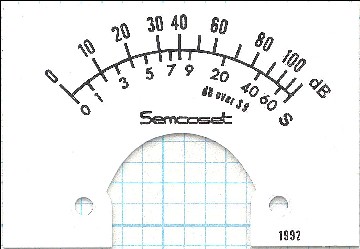The image features a background that resembles light teal graph paper, commonly used in math classes for graphing purposes. Overlaying the background is an intriguing object that could either be a piece of paper or plastic. The object is centrally positioned towards the bottom and it has a notched-out vertical section topped with a rounded dome. 

On both the left and right sides of this object, there are circular cutouts through which the graph paper is visible. Directly below the right circle is the year "1992." The top section of the object features a curved scale starting at 0, labeled with intervals of 0, 10, 20, 30, 40, 60, 80, 100, ending with the designation "dB," likely indicating decibels.

The bottom section showcases another scale starting at 0, labeled with intervals 0, 1, 3, 5, 7, 9, 20, 40, 60, and culminates in the character "S," though the significance of this "S" is unclear. Beneath the scale on the top section, there appears to be some mathematical or scientific notation which is difficult to decipher. Horizontal text below this notation reads "semicoset" or something similar. All the lines and text on this object are rendered in black.